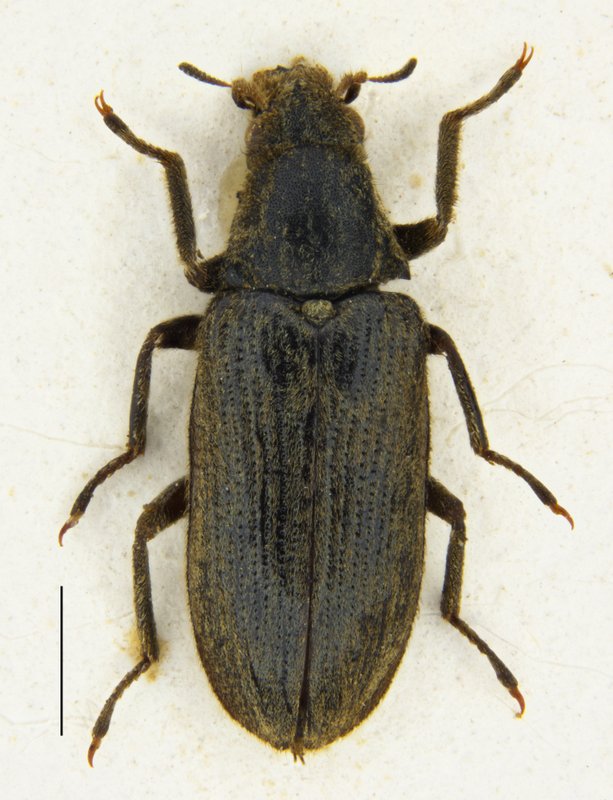This detailed photograph captures an extreme close-up of a bug, possibly a beetle or a cockroach. The bug exhibits a predominantly dark, almost black coloration with subtle brownish tints. It has six legs, three on each side; the front legs appear more prominent, and all legs seem to end in small claw-like structures. The insect's long, elongated body is slightly fuzzy, with noticeable fine hairs. Two thick antennae and two distinct eyes are visible, contributing to its detailed and somewhat unsettling appearance. The setting appears to be indicative of a display, likely in a museum, with the bug mounted vertically against a white background, possibly concrete. The image also includes a line on the lower left, perhaps serving as a measurement indicator for the display. The high magnification emphasizes the intricate textures and details of the bug's anatomy.